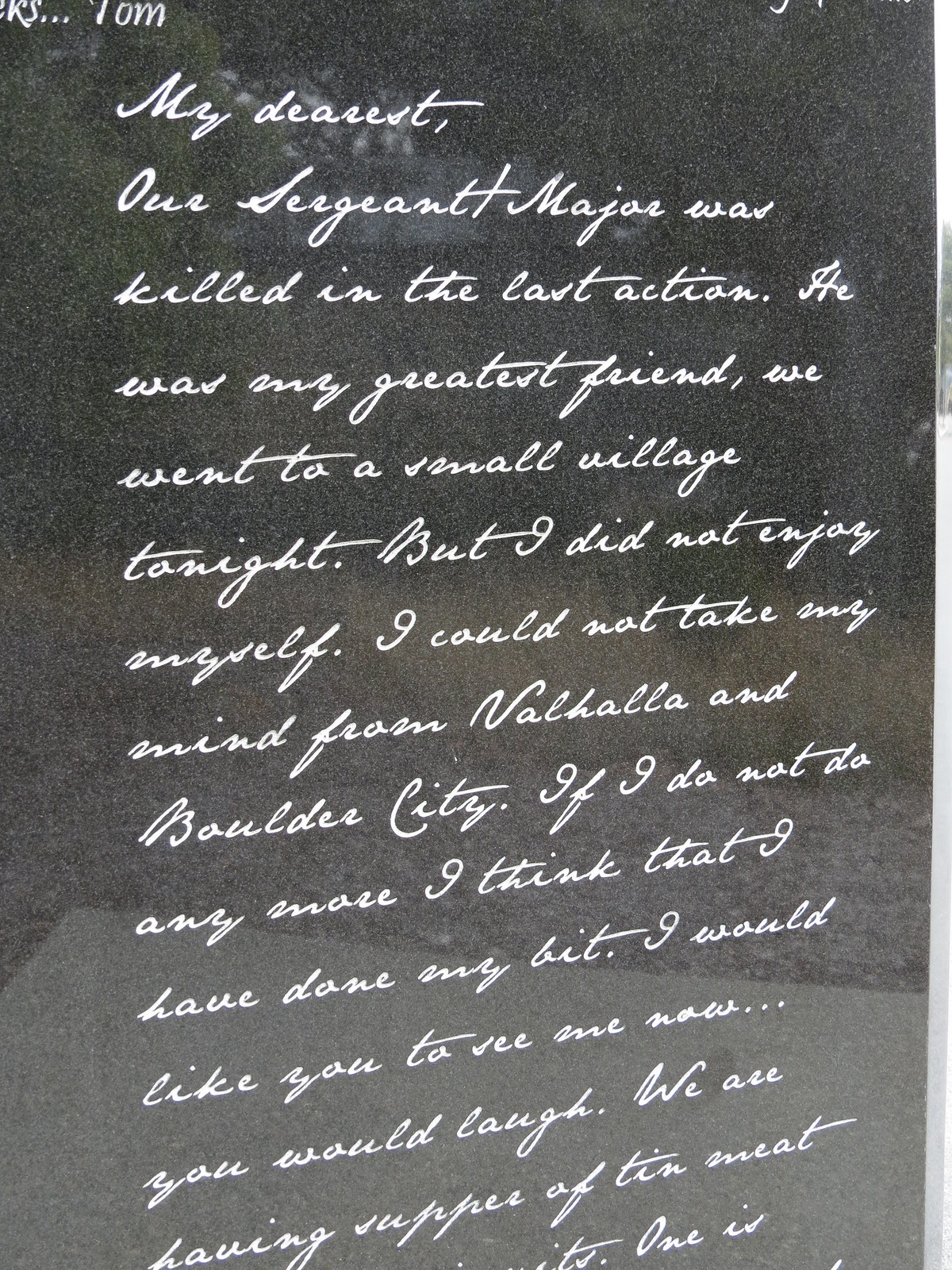The image depicts a skewed, photonegative-like scan of a handwritten letter with white cursive writing on a dark, almost black background. The top of the letter features partially visible letters "RS...". The readable portion of the letter starts with "My dearest," and continues, "Our sergeant major was killed in the last action. He was my greatest friend. We went to a small village tonight, but I did not enjoy myself. I could not take my mind from Valhalla and Boulder City. If I do not do any more, I think that I have done my bit. I would like you to see me now. You would laugh. We are having supper of tin meat." The text becomes unreadable afterward, with only the partial phrase "One is" decipherable at the very end. The background appears dark gray and granular, and the image is tilted, contributing to its skewed appearance. The overall lighting of the image is not optimal, making the details harder to discern.